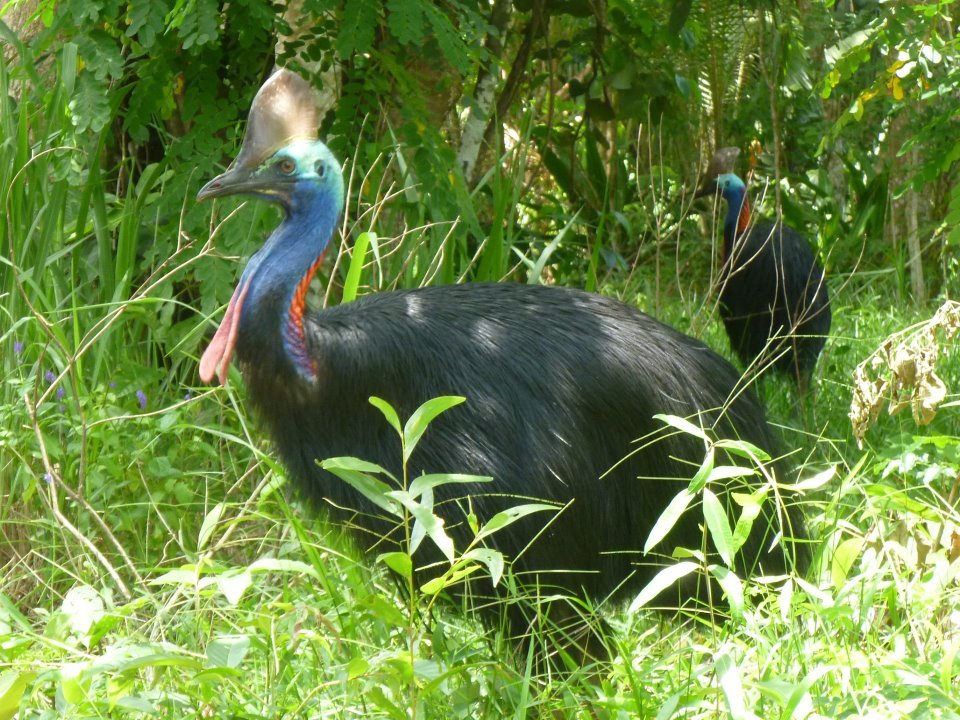The image, taken outdoors during daylight, captures a close-up view of a leafy wooded area in the background, with a foreground dominated by high and medium-high grass and foliage. At the center of the frame stands a large bird, resembling a peacock, with its head turned towards the left. It features a blue neck and head with a hint of red or pink on the back of its neck and a distinctive brown, helmet-like comb on top of its head. The bird's body is curved and covered in black feathers that appear more like hair. Its wings are closed. To the right, slightly trailing behind, is another similar bird. The scene, rich in greenery, is set in the shade, evoking a sense of wildlife and ornithology.